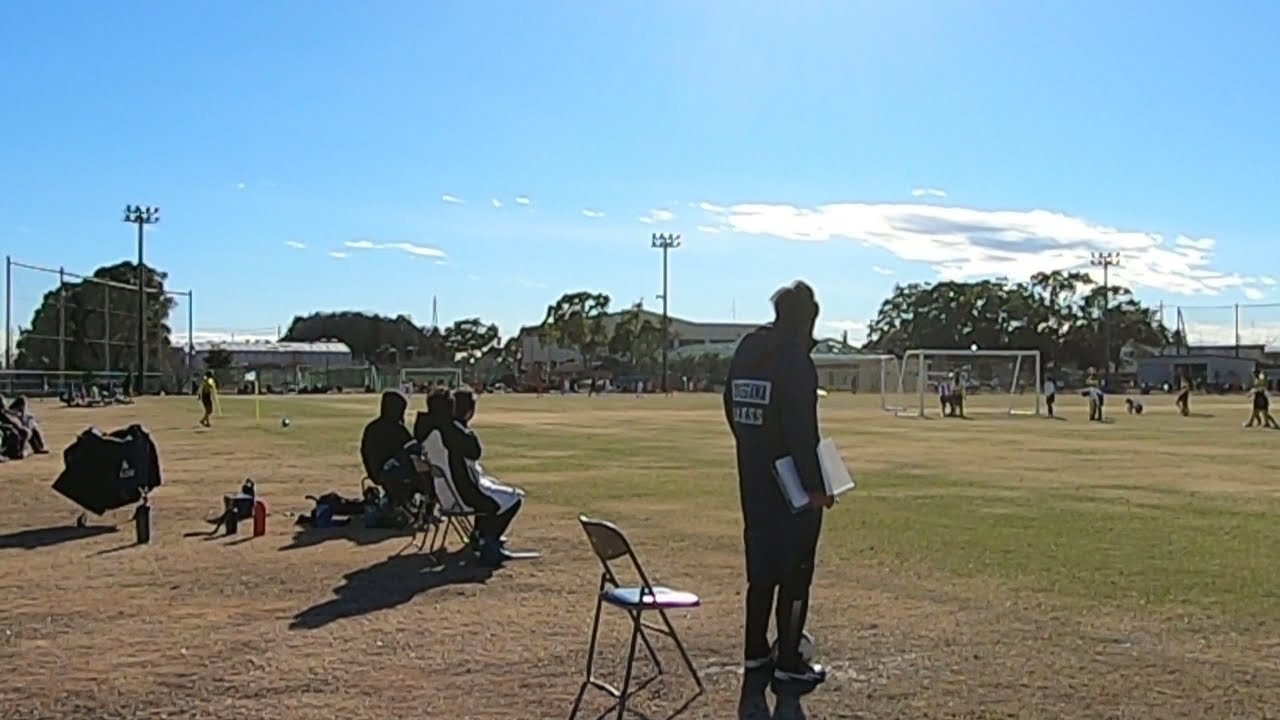The image depicts a full-color, horizontally rectangular photograph taken outdoors on a sunny, yet cool day at a soccer match, possibly involving high school or middle school players. The scene is set on a somewhat worn, patchy field with grass that varies in hues of green and brown, indicative of heavy use and perhaps insufficient watering.

Occupying the foreground, a coach stands on the sidelines, wearing a black tracksuit and holding a clipboard in his right hand. In front of him is a folding chair, where he was likely seated before. Several spectators sit in similar folding chairs nearby, all bundled up in coats and hoodies, suggesting the coolness of the day. Behind them, a few drinks and cups are set up, hinting at preparations for the game.

The sky is a brilliant blue with a swath of clouds to the right, and towering light poles stand above the scene, unlit due to the midday sun. In the background, players are seen either stretching or preparing for the match amidst a backdrop of homes, absorbing the anticipation in the air on this clear, picturesque day.